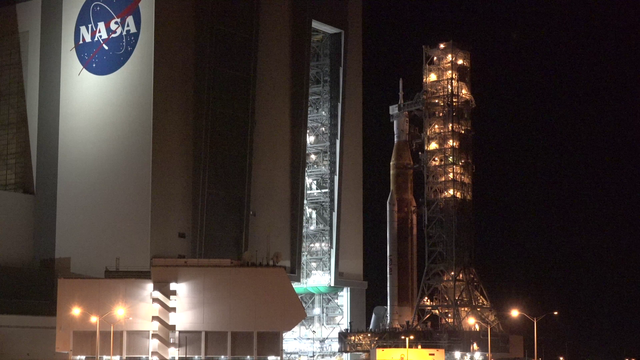The nighttime photograph captures a striking scene at a NASA facility. On the left half of the image stands a large cement building, prominently featuring the illuminated blue NASA logo with its iconic white lettering and red vector symbol, all set against a dark sky. This building's open area suggests space for moving infrastructure necessary for rocket launches. To the right of this structure, a towering metal scaffolding, brightly lit throughout, extends higher than the adjacent rocket. The spaceship itself features a white tip, progressing to a broader golden hue towards its base. Two street lamps at the bottom frame the scene, one on each side, further illuminating the setup and highlighting the intricate details of this impressive nighttime snapshot.